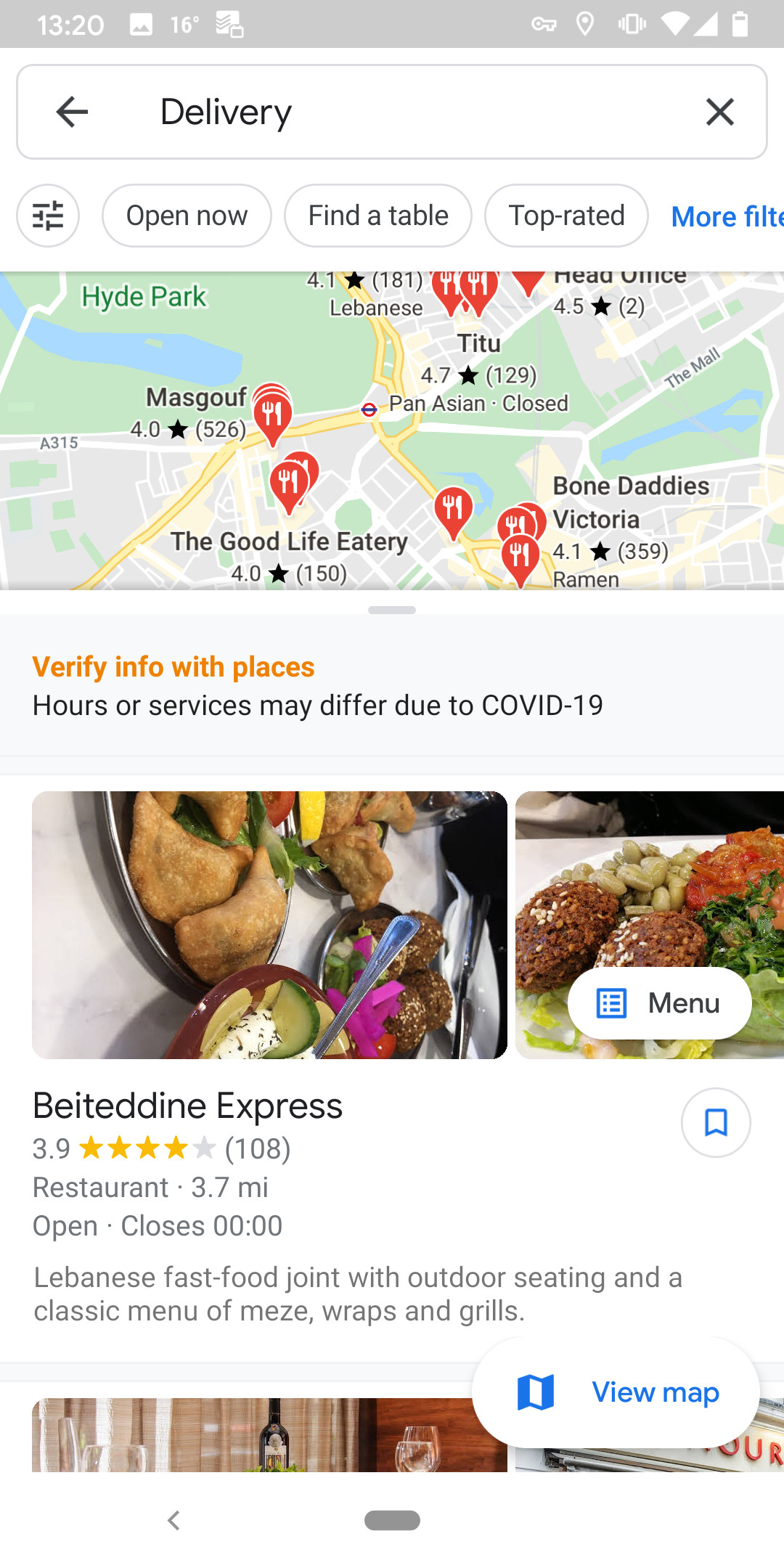**Descriptive Caption:**

The image appears to be a screenshot from a tablet or smartphone, as indicated by certain visual elements. At the top, the dark gray bezel shows "13:20" in bold white text, signifying military time. Below that, a white square icon with black mountains suggests a standard screenshot notification typically seen on mobile devices. The temperature is displayed as "16 degrees."

On the top right corner, there are various notification icons including a key, a map pin, a vibrating arm, a vibrating phone, a wireless signal indicator, and a nearly full battery. The search bar, which is rounded and dark gray, features a black left-pointing arrow, the word "delivery" centered, and a black "X" on the right side.

Underneath the search bar, clickable buttons are visible. The first button displays a white circle with sporadic black lines, while the subsequent sub-buttons include "Open now," "Find a table," "Top rated," and partially visible hyperlinked text "more filters." Red pins are clustered on what appears to be a map, each with a fork and knife symbol, suggesting restaurant locations based on the search term "delivery."

The text "Verify info with places" is in gray, followed by a note in black: "Houses or services may be different due to COVID-19." Various close-up food images are shown: a plate with golden-brown breaded chicken, avocados, white topping likely sour cream, and possibly ice cream dusted with chocolate and garnished. 

On the right side, another food image depicts a brown Salisbury steak, with crispy potatoes, diced tomatoes, and garnished with dark and light green leaves. Further down, a restaurant listing for "BETD Express" is highlighted in black bold text with a gray 3.9 out of 5-star rating (stars in gold) and "108 reviews" in parentheses. The listing includes a bookmark icon in a white circle bordered in dark gray, with a dark green or blue bookmark symbol. 

Below the rating, the text describes the restaurant as a "Lebanese fast food joint with outdoor seating and a classic menu of MEZE, wraps, and grills.” It notes a distance of "3.7 miles" and its open status. Adding to the visual detail, there's another photograph against a tan wall with a red wall adjacent, and an oval white button with a blue movie-like map symbol labeled "View map" in bold blue.

Finally, the screenshot's bottom bezel is small, oval, and dark gray, hinting at navigation controls.